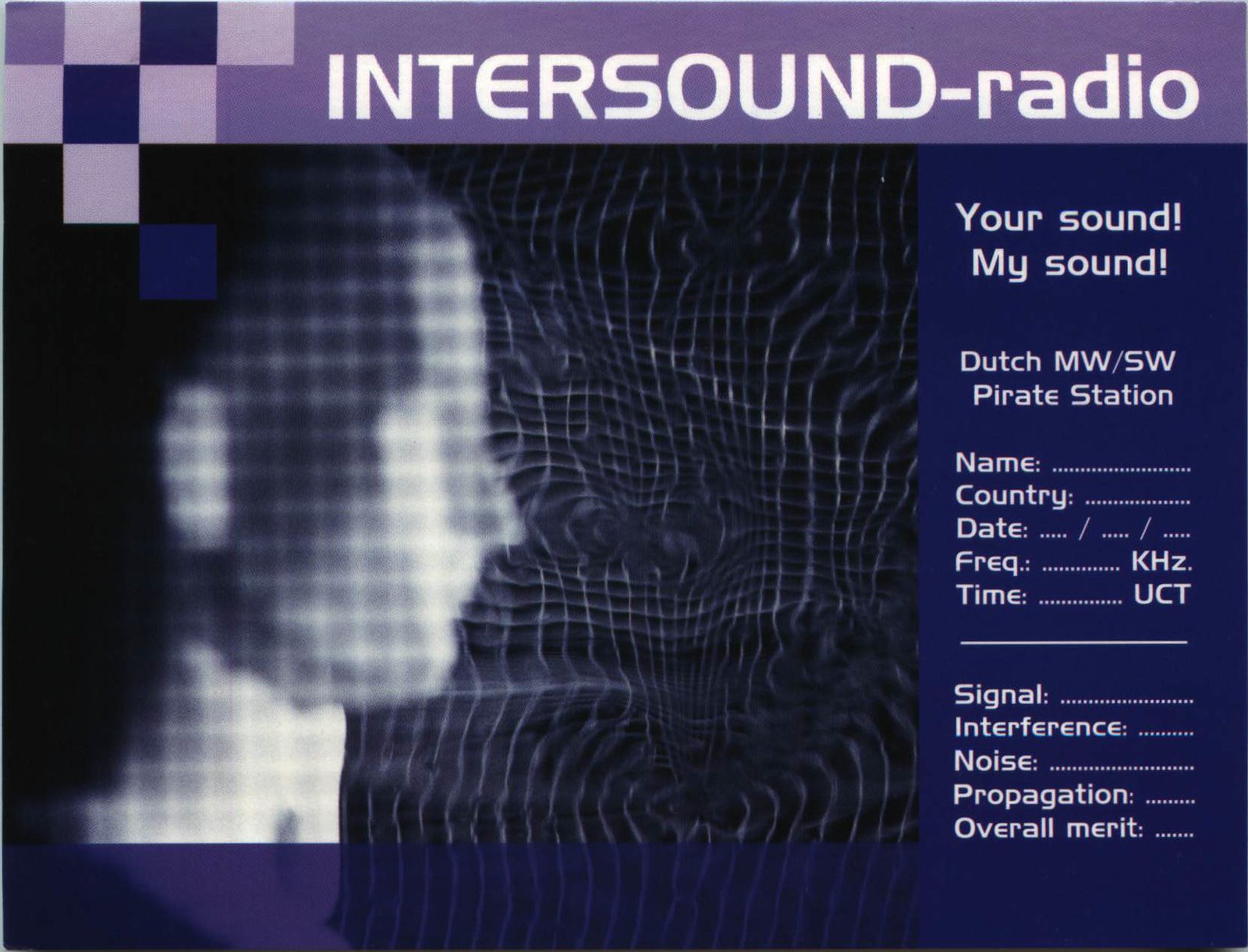The image is a visually striking postcard titled "Intersound Radio," characterized by its futuristic and graphic design elements. Centrally, it features the profile view of a white, mannequin-like figure with a light grid projected onto it, symbolizing sound waves and frequencies. This central figure is surrounded by a wavy grid and the entire composition sits against a vivid purple background with large, pixel-like squares on the left. At the top of the postcard, the title "Intersound Radio" is prominently displayed in white text on the purple banner.

To the right of the mannequin figure, a dark blue vertical bar contains white text in a vertical layout reading, "Your Sound, My Sound, Dutch MW/SW Pirate Station." Below this, several blank fields are listed to capture details such as name, country, date, frequency (in kilohertz), time (in UCT), along with sections to evaluate signal, interference, noise, propagation, and overall merit. The overall aesthetic resembles a high-tech, media-centric advertisement or form, intertwining both artistic and functional elements.